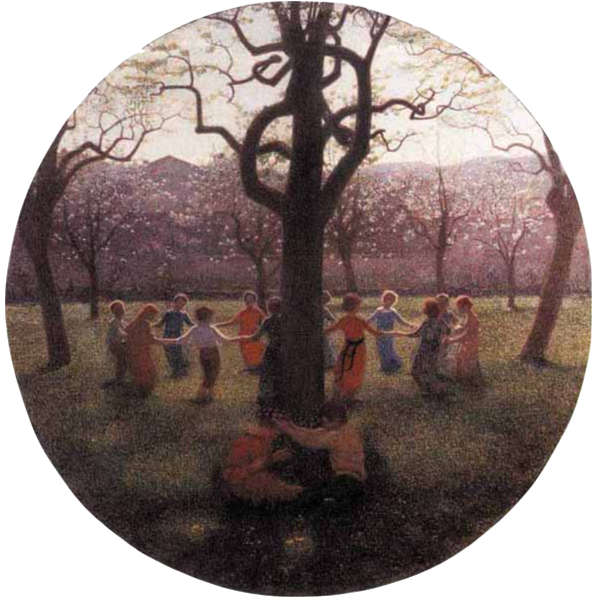The image is a round, medieval-style painting that features a central large black tree with curly, leafless branches, suggesting early spring as buds begin to form. The tree, which resembles an oak, is set against a park-like background filled with children playing. In the foreground, two children sit at the base of the tree, one facing left and the other facing right, with the boy on the right extending his hands as if placing something on the other child's head. Surrounding this central tree, a group of about 12 or 13 children, boys and girls in multicolored clothing including red and blue dresses and a boy in a white shirt with brown pants, form a ring by holding hands, likely engaged in a game such as “Ring Around the Rosy.”

To the sides of the central tree, two other leafless trees with curly branches lean outward—one to the left and the other to the right. In the distance, a row of smaller trees adorned with white flowering blossoms extends across the background, adding a delicate contrast to the bare trees in the foreground. Beyond this floral line, hills or mountains rise in the further background. A subtle hint of a house appears on the far left edge of the image, adding depth and a sense of place to the idyllic, bucolic scene.